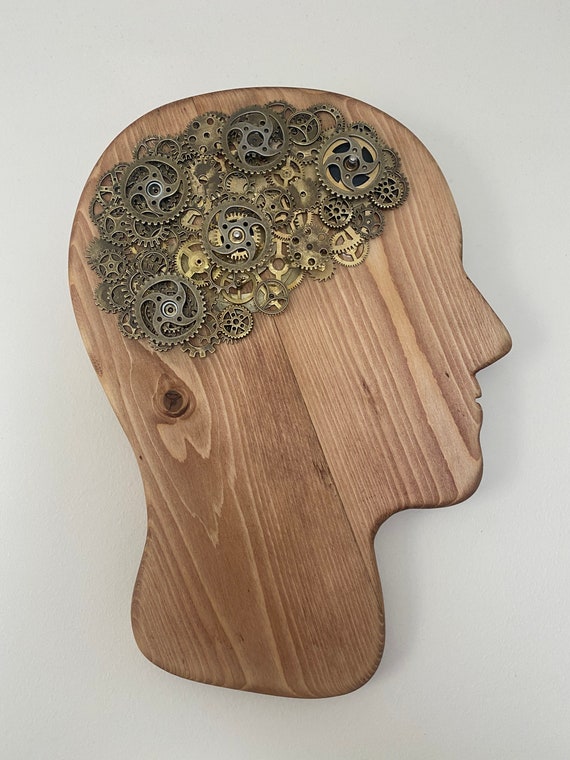The product photograph showcases a wooden plaque, elegantly displayed on a flat white surface to emphasize the product for online commercial purposes such as shops, catalogs, and websites. The plaque is crafted from light brown wood with distinct wood grain running diagonally from the top left to the bottom right. It is cut into the silhouette of a person's head, facing right, clearly outlining the mouth, nose, eyes, and neck. Prominently, where the brain would be, multiple metallic cogs and gears, colored in brass, gold, and copper, are intricately arranged. These gears, varying in size and shape—with some as large as quarters and others as small as pennies—are meticulously stacked on top of each other, filling the entire brain area. The photograph captures the detailed textures of both the wood and the metal components, making the product stand out against the stark white background.